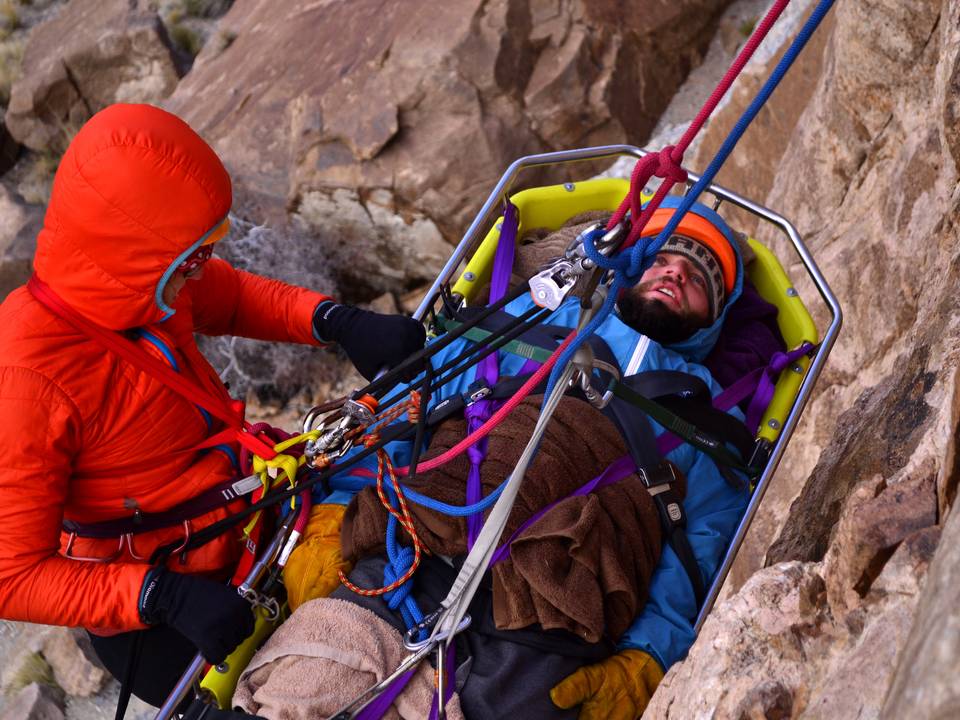This is a color photograph depicting a dramatic mountain rescue operation on a steep, jagged brown and gray rock face. At the center of the image, a man lies flat in a silver metal stretcher, secured with multiple black and pink straps crisscrossing over him. He is wearing a blue jacket with a blue hood, an orange cap peeking underneath, orange-brown gloves, and has a black-brown beard and mustache. On top of him is a dark brown towel.

The stretcher is connected to a system of red, blue, and pink ropes and pulleys that extend upward and out of the frame, giving the impression that he is being hoisted up the rock face. Surrounding the man are numerous jagged rocks in varying shades of light brown to dark brown and light gray.

To the left of the stretcher, assisting in the rescue, is a person dressed in a bright orange hooded jacket with black gloves, black pants, and a black harness roped into the system. The person appears to be wearing glasses, and the jacket features a blue line around the hood’s edge and a blue zipper. This rescuer is firmly holding onto the side of the stretcher, ensuring the man's stability as they both ascend the vertical cliff face in what looks like a coordinated, life-saving effort.